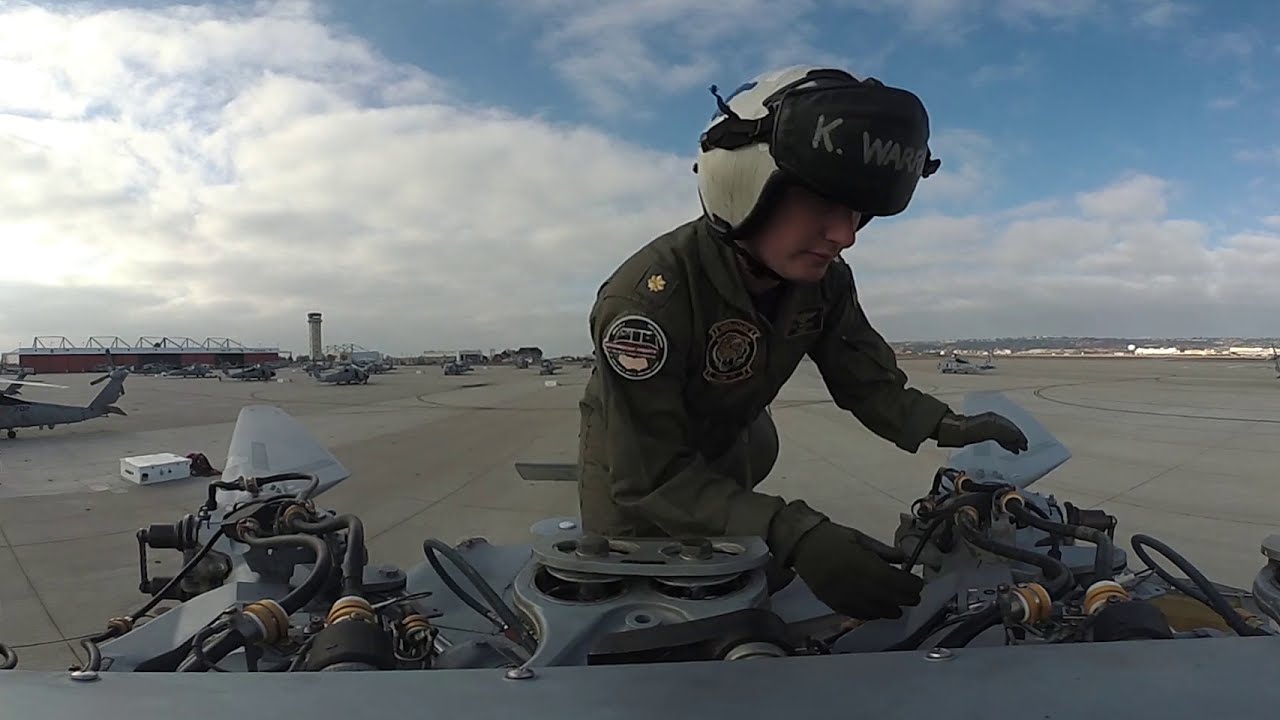The image features a figure dressed in an olive green jumpsuit, covered with various sewn-on badges and patches, who appears to be a member of a military or police force. The individual has a white helmet emblazoned with the letters "K.W.A.R.", though the meaning or full text remains unclear. Dark gloves cover their hands as they lean over and pour something into a mechanical device or engine that spans horizontally across the frame. The device is detailed with black hoses and a grayish metallic finish. The person’s side profile reveals them to be white. The setting is expansive and flat, resembling an airport tarmac or a large military base, with light gray surface and numerous helicopters and airplanes parked in the background. The sky, occupying nearly half of the image, is clear with a few white clouds, setting the scene in an open and likely secure area. Additionally, a substantial hangar building can be seen on the left, adding to the sense of a designated aviation or military zone.